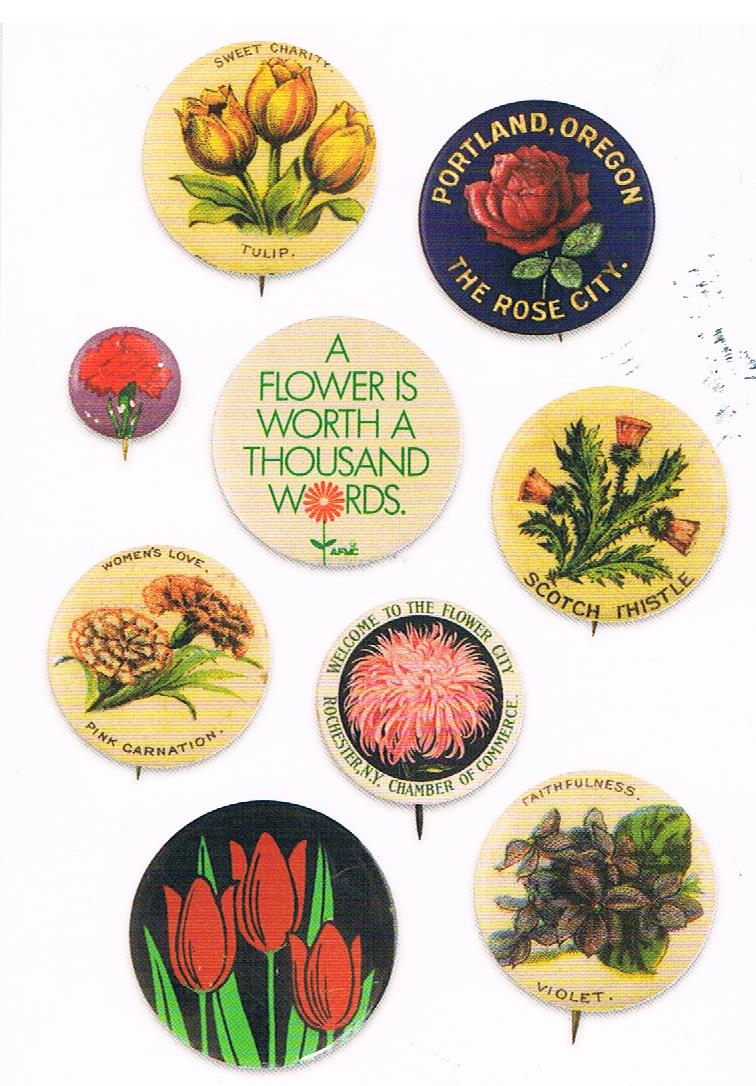The image shows a collection of circular stickers or signs, presumably meant for gardening or decorative purposes, each featuring different flowers and associated text. The sizes of these items are indeterminate as there is no scale reference.

1. One sticker features **yellow and red tulips** with the text "Sweet Charity Tulip" at the bottom. It’s a drawing rather than a photograph.
2. Another sticker, with a **blue background**, has the text "Portland Oregon the Rose City" in yellow, accompanied by a red rose illustration.
3. A small purple sticker shows **red flowers**, though it remains unidentified by text.
4. A brown background sticker with green text reads "A flower is worth a thousand words," featuring a red flower.
5. A **yellow circle sticker** shows **orange-colored scotch thistles** with green leaves, labeled "Scotch Thistle."
6. Another sticker, on a yellow background, displays **yellow and orange carnations** with "Women's Love Pink Carnation" written above them.
7. An additional sticker has a large, fluffy pink flower on a black background, bearing the text "Welcome to the Flower City Rochester New York Chamber of Commerce."
8. There’s also a sticker with a **black background**, displaying a cartoonish depiction of either red roses or tulips with green leaves.
9. The final sticker reads "Faithfulness," featuring **violets** in rich, deep purple with green leaves against a light brown background beneath the word "Violet."

All of the illustrations are more stylized drawings than hyper-realistic images.